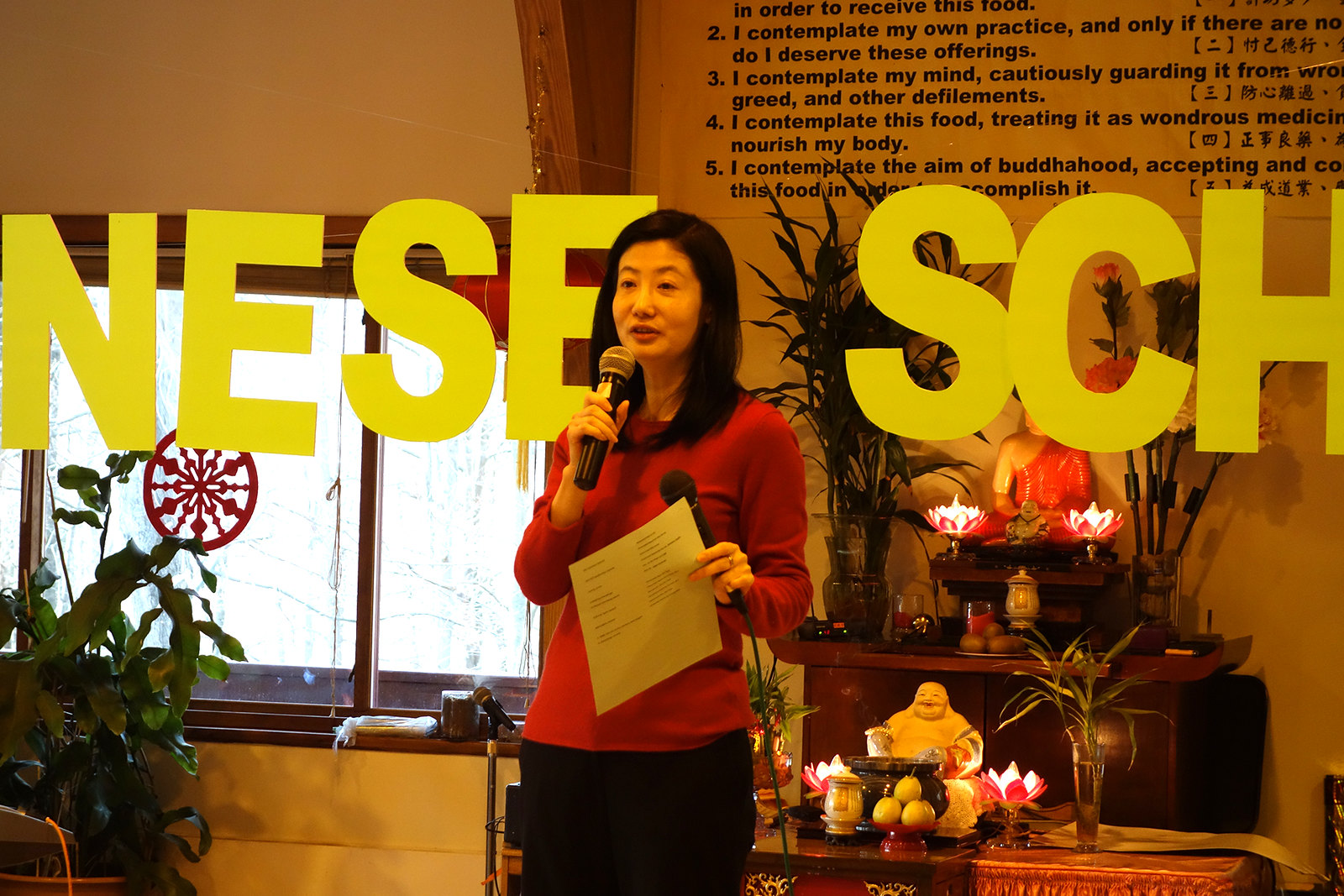In this indoor photograph, likely set in a Chinese school, a woman of Asian descent is standing prominently in front of an altar. She holds a microphone in one hand and a piece of paper in the other, delivering what appears to be a talk or presentation. The woman, who has shoulder-length black hair, is dressed in a long-sleeved red top and black bottoms. Behind her, large yellow letters partially spelling "N-E-S-E" and "S-C-H" suggest an educational setting. 

Central to the background is an elaborate altar dedicated to Buddha, featuring two distinct Buddha statues. The lower statue, recognizable by its joyful demeanor, is the Laughing Buddha, surrounded by lotus candles, possibly jade objects, and attractive foliage including plants in vases. Above this, another Buddha statue dressed in an orange robe graces the upper layer, also accompanied by candles.

Behind the altar, a piece of paper hung on the wall contains both English phrases and their Japanese equivalents. One discernible line reads, "Contemplate the aim of Buddhahood. Accepting this food in something, accomplish it." The entire setup emphasizes a serene and contemplative atmosphere, blending elements of religious reverence with an educational context.